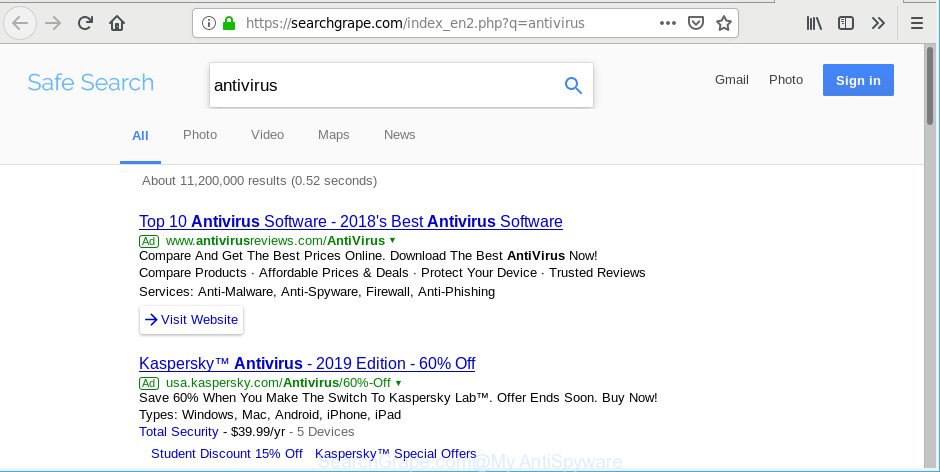This is a screenshot of a search results page from searchgroup.com. At the very top, the URL bar prominently displays "searchgroup.com." Directly below it, there's a grey bar. On the left side of this grey bar, the logo "SafeSearch" is displayed in blue.

In the center of this grey bar is the search bar, populated with the query "Antivirus." A blue magnifying glass icon is situated to the right of the search bar. Adjacent to this, there are options labeled "Gmail," "Photo," and a blue "Sign In" button.

Below this section is the top menu with the options: "All," "Photo," "Video," "Maps," and "News." The "All" option is highlighted in blue and underlined.

The main body of the page shows two search results. The first result is titled "Top 10 Antivirus Software 2018's Best Antivirus Software," and the second is "Kaspersky Antivirus 2019 Edition, 66% off." Both results are marked as ads, indicated by a green label "Ads" underneath the titles. Each result displays its respective URL in green, followed by a snippet of black text on a white background.